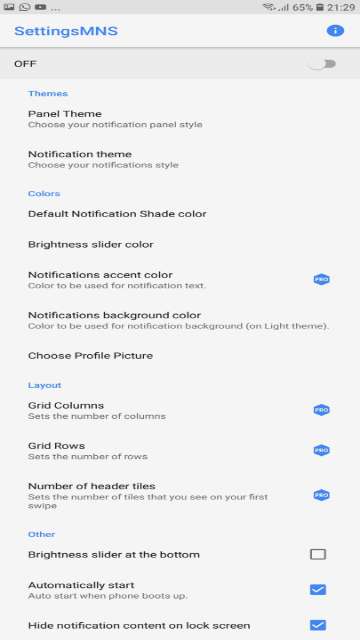### Detailed Image Caption

In this image, captured from a smartphone screen with a grey background, various elements are visible. At the top of the screen, several icons are displayed: WhatsApp, Screenshots, and YouTube, along with the Wi-Fi signal, network signal strength, and battery percentage, which is at 65%. The time on the device is shown as 21:29.

The open application on the smartphone screen is the "Settings" page, indicated by the word "Settings" written in blue at the top, followed by "MNS" and a blue exclamation mark to the right. Below this heading, there is a toggle switch that is currently turned off, with the label "Off".

The page is organized into several sections with blue subheadings. The first section is titled "Themes", with the subsection descriptions written in black text:
- **Panel Theme:** Choose your notification panel style.
- **Notification Theme:** Choose your notification style.
- **Colors:** Options to customize the default notification shade color, brightness, light shade color, notification accent color, notification text color, and the notification background color for the light theme.

There is an additional option to choose the profile picture linked to notifications.

Another section is titled "Layout", but it is noted that the layout features are only available in the Pro version of the app. This section includes:
- **Grid Columns**
- **Grid Rows**
- **Number of Header Tiles**

There is a green square labeled "Pro" beside the Layout heading, indicating these features are part of the professional version.

The final section is labeled "Other", which includes:
- **Brightness slider at the bottom:** This option is not checked.
- **Automatically start:** This setting is checked.
- **Hide notification content on lock screen:** This setting is also checked.

In this context, the blue color is used for check marks and other interactive elements, including the switches and toggles on the screen.